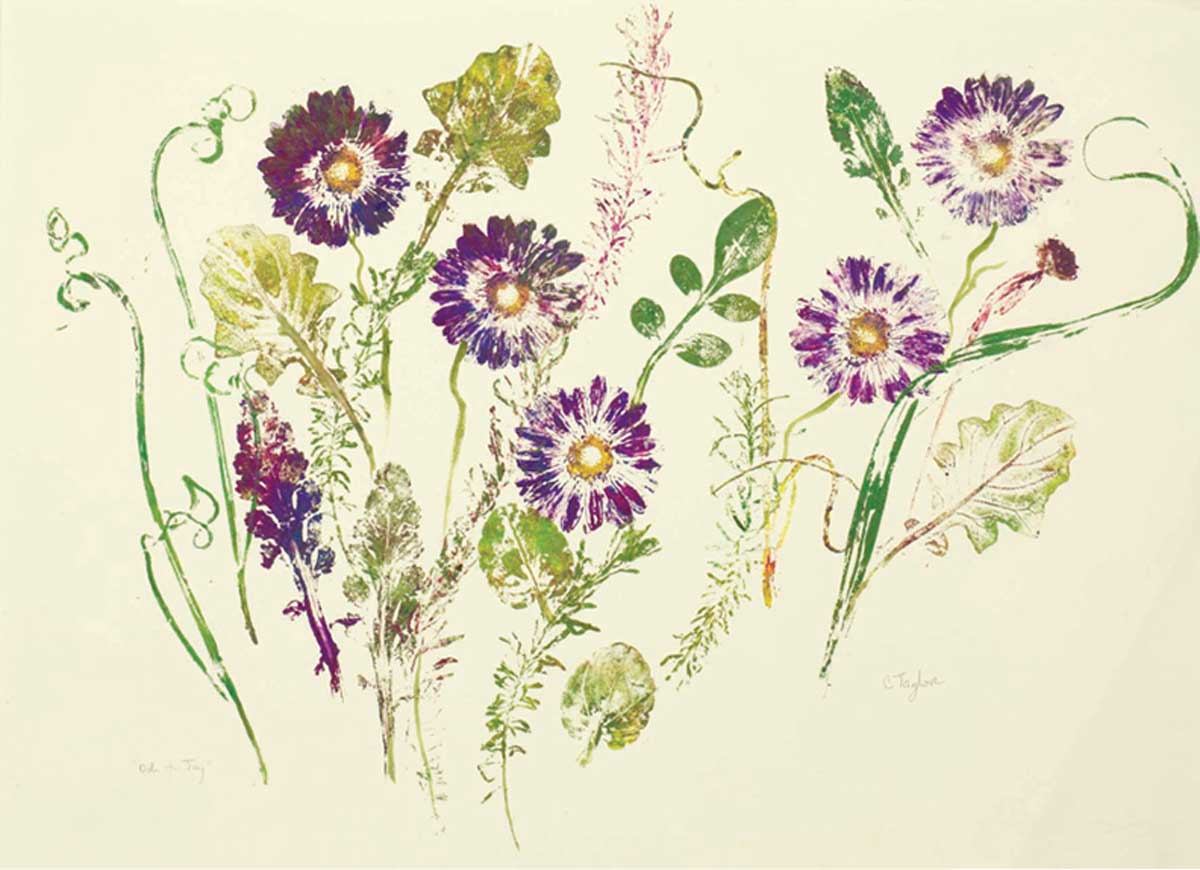This image is an artist's print of a detailed painting depicting a series of wildflowers against a light gray, creamy canvas. The composition features a close-up view of the flowers, highlighting their intricate details. Central to the image are the main flowers, primarily in deep purples outlined with lighter hues, centered around golden yellow buds. These flowers extend from green stems and are complemented by scattered green leaves and additional miscellaneous stems. In the bottom left corner, a solitary purple flower stands out, differing slightly in design from the rest. The artwork gives an impression of either pressed flowers dipped in paint or a carefully curated painting technique, creating a textured look with some areas appearing rough and faded. Notably, the image also includes what could be signatures, with "C. Taylor" possibly inscribed on the right side.